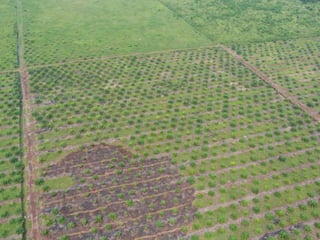This aerial image captures a segmented farmland divided into four quadrants. From this high vantage point, the details of each quadrant are subtle and indistinct. The predominant color across the image is green, likely representing grass or various crops. The lower half of the image features parallel rows of brown soil, suggesting newly planted crops, though the specifics are indiscernible from this height. On the left and right sides of this section are elongated, brown pathways that could be dirt roads or dividers for irrigation purposes. The bottom-left corner showcases a large patch of exposed soil with faint lines, indicative of a garden or a prepared field area. Towards the back of the image, there is a more uniform expanse of green, possibly a simple field of grass. Overall, the image presents a patchwork of different shades and textures, hinting at a variety of agricultural activities or plantings across the landscape.